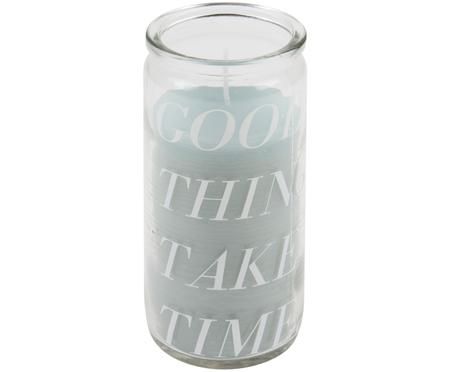The image showcases a cylindrical, clear glass candle centered perfectly in the frame against a white background, illuminated in bright, solid lighting. The candle wax inside the glass container is a soft, light blue, almost mint green in hue, with a thin white wick extending from it. The wax fills approximately four-fifths of the container, up to the word "GOOD" in the text. The white, uppercase text on the glass reads, "GOOD THINKING TAKES TIME," with each word placed on its own row. The glass container also features a lip at the top and appears darker at the bottom, giving the image a sense of depth and clarity. The candle is new and unlit, emphasizing its pristine condition and detailed craftsmanship.